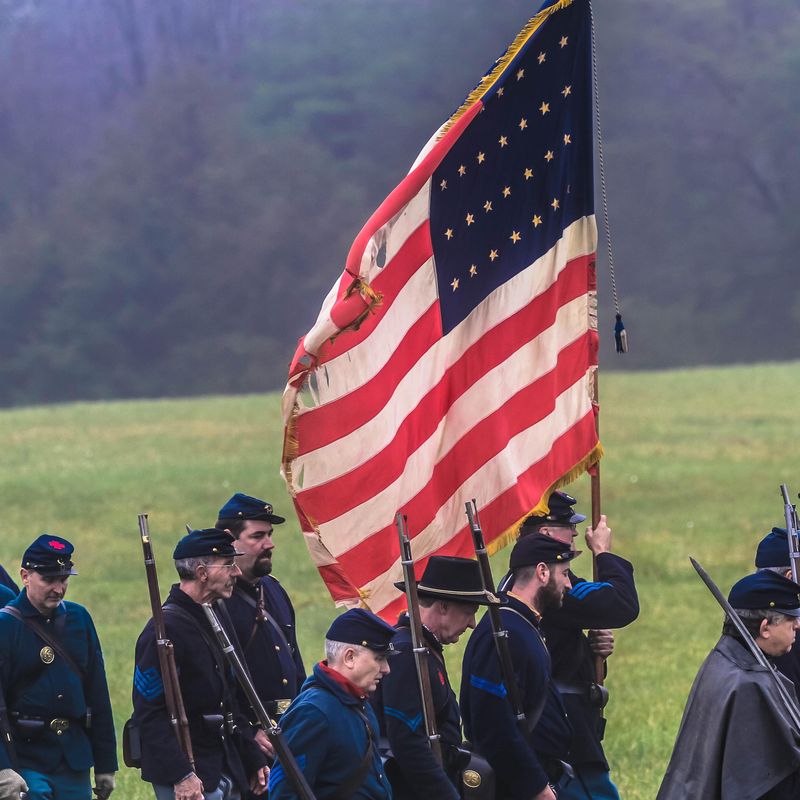The image is a color photograph taken outdoors during the daytime in a foggy or possibly rainy setting. The gloomy, dim lighting contributes to a historical atmosphere. In the foreground, a group of nine middle-aged to older men march in rows, all dressed in the dark navy blue uniforms and caps typical of Union soldiers from the American Civil War era. These reenactors are engaged in a Civil War reenactment event, portraying the Yankee soldiers of the Union Army. At the center of the formation, one man prominently holds a large, weathered American flag, the red and white stripes billowing to the left and the blue field with white stars positioned in the upper right corner. Each soldier carries a musket over his right shoulder, adding to the authenticity of the scene. The background features a grassy field leading to mist-shrouded hills and possibly a wooded area, enhancing the vintage ambiance of the photograph.